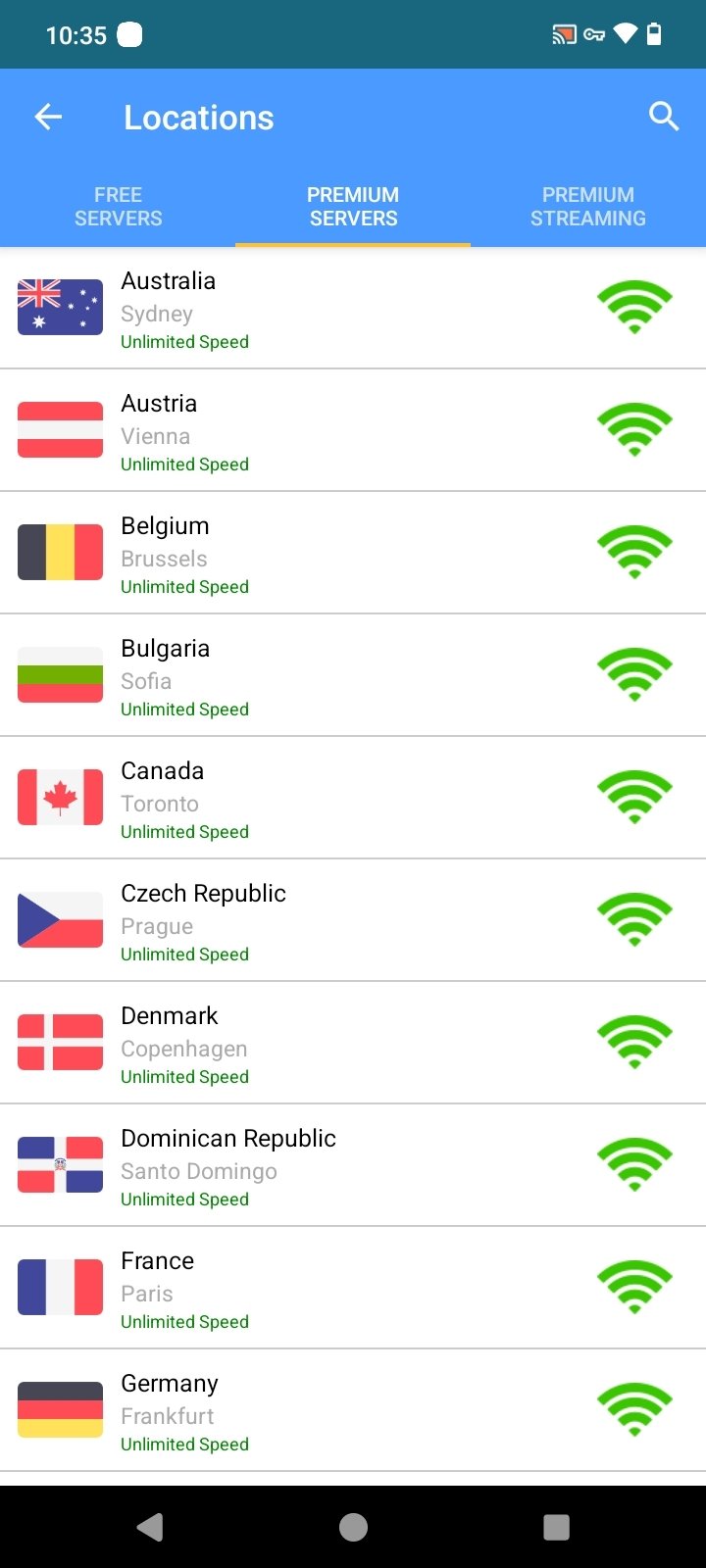The image displays a smartphone screen with a status bar at the top. The time is shown as "11:22," accompanied by an icon of a bell with a diagonal line through it, indicating that notifications are muted. Next to the bell icon, there is a full battery icon. Below the status bar, within a black rectangular box, the text "Privacy Policy" is prominently displayed. The privacy policy text begins about three inches below this header, consisting of four to five paragraphs detailing the information.

A subheading after these paragraphs reads "Information Collection and Use." Directly beneath this subheading, five circles are aligned vertically, each associated with a specific service: "Google Play Services," "AdMob," "Google Analytics for Firebase," "Firebase Crashlytics," and "Facebook." These service names are written in blue text next to their corresponding circles.

Further down, to the left in black text, is the heading "Log Data." At the very bottom of the image, there is a long black rectangle. Inside this rectangle, there is an arrow pointing left, a gray circle in the center, and a gray square to the far right.